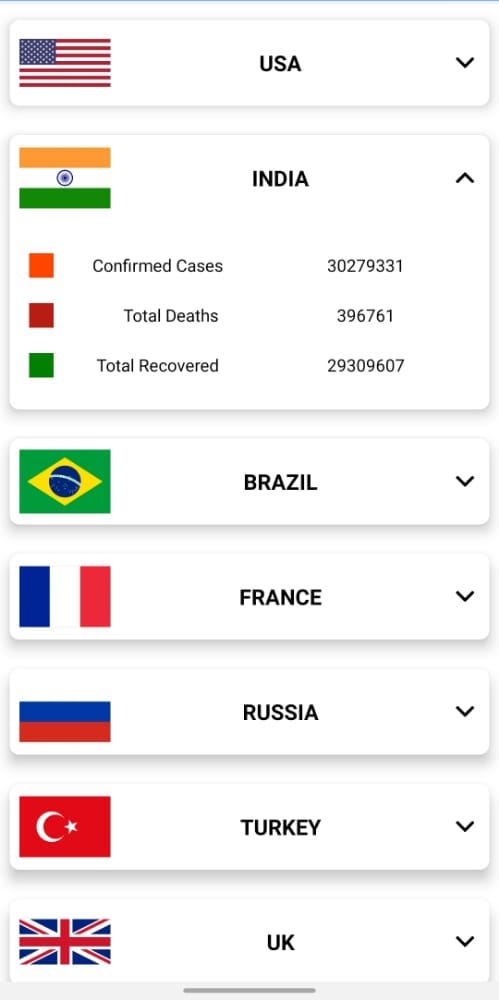The image is a screen capture displaying statistical data about various countries, likely related to a health outbreak such as COVID-19. At the top, there is a thin blue line. Below it, a series of white boxes with black text and country flags are lined up in a vertical sequence.

- **United States:** The American flag, featuring red and white stripes with white stars on a blue field, is displayed. The box includes data such as confirmed cases, total deaths, and total recovered. The confirmed cases are indicated with a red box, total deaths with a darker red box leaning towards maroon, and total recovered with a green box.

- **India:** The Indian flag, showcasing horizontal stripes of orange, white and green with a blue Ashoka Chakra in the middle, is displayed. The same categories of data are shown: confirmed cases in a red-orange box, total deaths in a dark red box, and total recovered in a green box.

- **Brazil:** The Brazilian flag is shown, with its green field, yellow diamond, and blue globe with stars at the center.

- **France:** The French flag, featuring vertical stripes of blue, white, and red, is displayed.

- **Russia:** The Russian flag is shown, with horizontal stripes of white, blue, and red.

- **Turkey:** The Turkish flag, a red field with a white crescent moon and star, is displayed.

- **United Kingdom:** The UK’s Union Jack, a mix of red, white, and blue crosses, is featured.

Below these flags and data boxes, there is a thin gray line and a gray box. The text in the boxes is in bold, black font and is very easy to read against the white background. The image quality is clear and detailed. While not explicitly stated, the statistics suggest the image is likely related to a COVID-19 dashboard or another health outbreak monitoring tool.